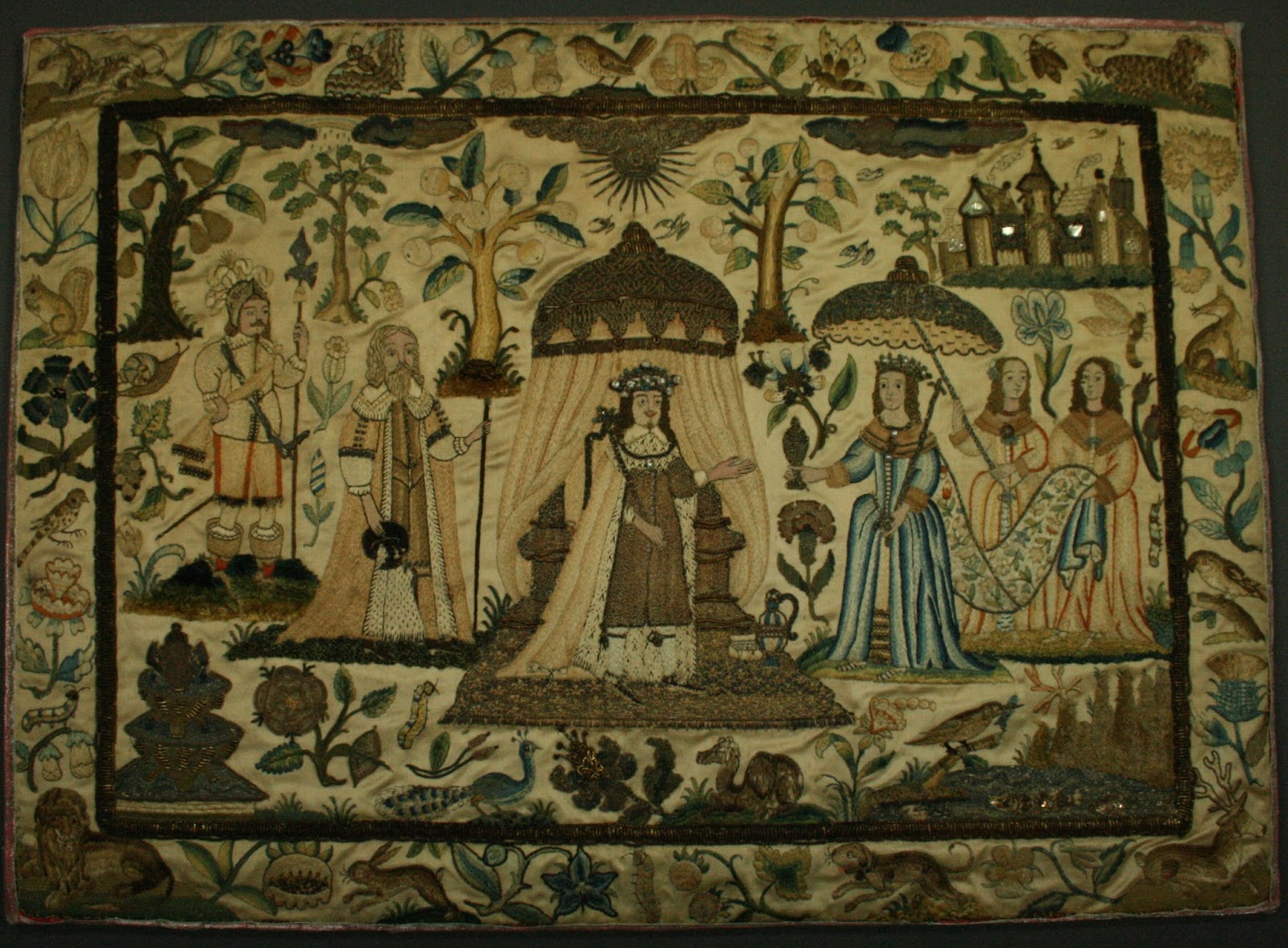This intricate and stylized artwork, possibly a medieval tapestry or an ancient painting, depicts a scene rich in historical and cultural detail. The border is lavishly adorned with a menagerie of animals and plants, including rabbits, felines, birds, dragons, foxes, squirrels, and various flowers, all intricately woven or painted. Central to the composition are figures that evoke a scene of Middle Eastern royalty or perhaps Biblical characters. A king, donning a flowing cape and crown, stands alongside a queen in a blue dress, her train held by attendants. Both are shaded by ornate umbrellas. Surrounding them are several other figures: perhaps an advisor, a knight akin to those seen in Spanish depictions, and servants who hold significant items, including a cross. In the backdrop, ancient tents with domed tops add an Egyptian flair, and a small castle or church is nestled amidst an abundance of trees. The overall palette of the artwork consists of rich greens, browns, and tans, with notable blue accents in the dresses. This piece is a tapestry of history and nature, interweaving various elements to create a scene steeped in tradition and storytelling.